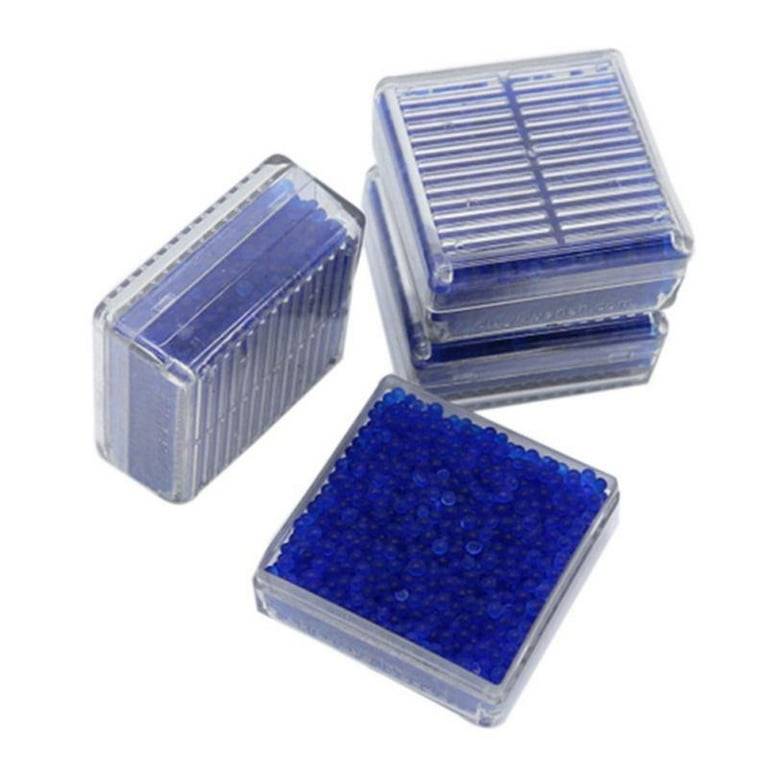The image features four clear plastic containers, each resembling small pencil cases, filled with bright blue, very small beads. These beads are slightly translucent and opaque, almost the size of salt grains. In the top section of the image, two or three of these containers are stacked on top of each other, securely closed yet still revealing the vibrant blue beads inside. On the left side, another container stands upright, allowing a clear view through its plastic, holographic material. At the bottom, a square-shaped plastic container lies open, fully displaying its contents of tiny blue beads against a white background. None of the containers appears to have any beads spilling out.